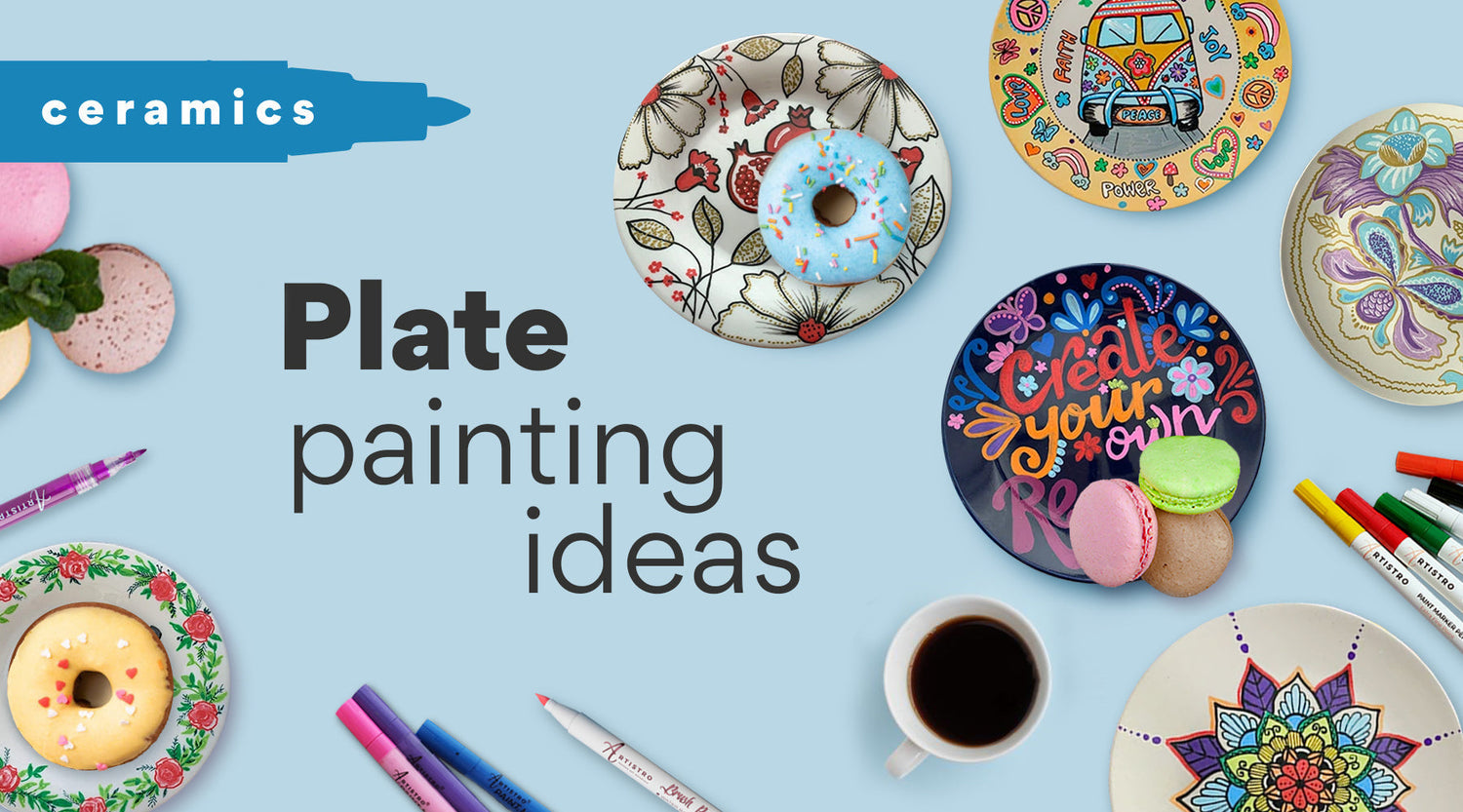The image features a light blue background with a darker blue highlight bar shaped like a marker in the top left corner, containing white text that reads "Ceramics." Below this, centrally located in black writing, are the words "Plate Painting Ideas." Scattered around the text are various design elements, including five detailed plates on the right side. These plates showcase an array of artistic designs: one with a white flower painted on a white background alongside a blue donut, another dark-colored plate with bright floral patterns and macaroons, and a particularly eye-catching plate depicting a Volkswagen bus with peace signs, rainbows, and encouraging words like "Faith" and "Joy." One of the plates invites creativity with the phrase "Create Your Own Plate," and another displays pastel colors with a peach-colored donut. Adding to the artistic theme, several markers are placed around the plates, and a cup of coffee is situated toward the bottom center, enhancing the creative and cozy atmosphere of the scene.